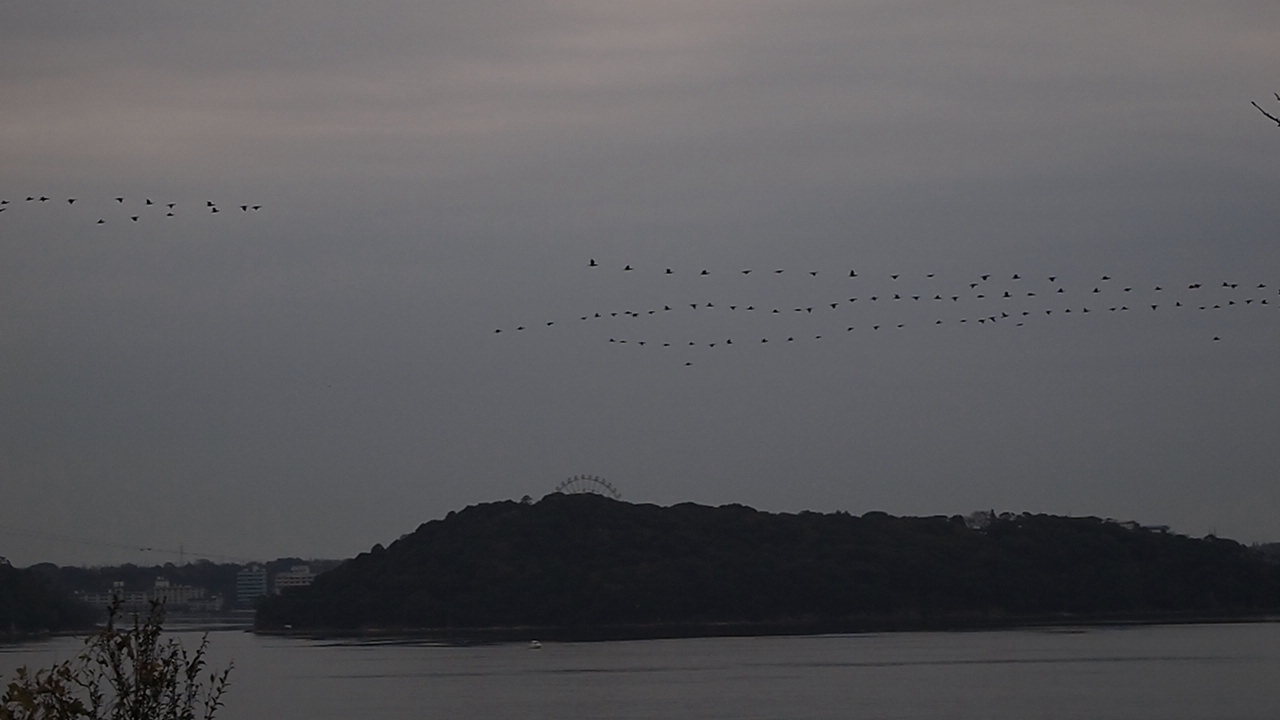The image captures a serene yet dramatic natural scene taken from the edge of a river at dusk. The sky is overcast, making it so cloudy that no trace of the sun is visible, casting a dark, somber tone over the landscape. In the sky, two prominent groups of birds fly in large, long V patterns, adding dynamic movement to the composition. Beneath them lies a still, calm body of water, reflecting the darkened sky. At the center of the image is a silhouette of a large island adorned with the outlines of trees, bushes, and shrubs, all merging seamlessly into the shadowy contours of a significant hill. Behind this landmass, the very top of a grand Ferris wheel peaks out, suggesting the presence of an amusement park. To the left of the Ferris wheel, distant buildings hint at a small city or town on the far coastline. The picture’s overall darkness and cloudy atmosphere emphasize the tranquil yet mysterious beauty of nature at the twilight hour.